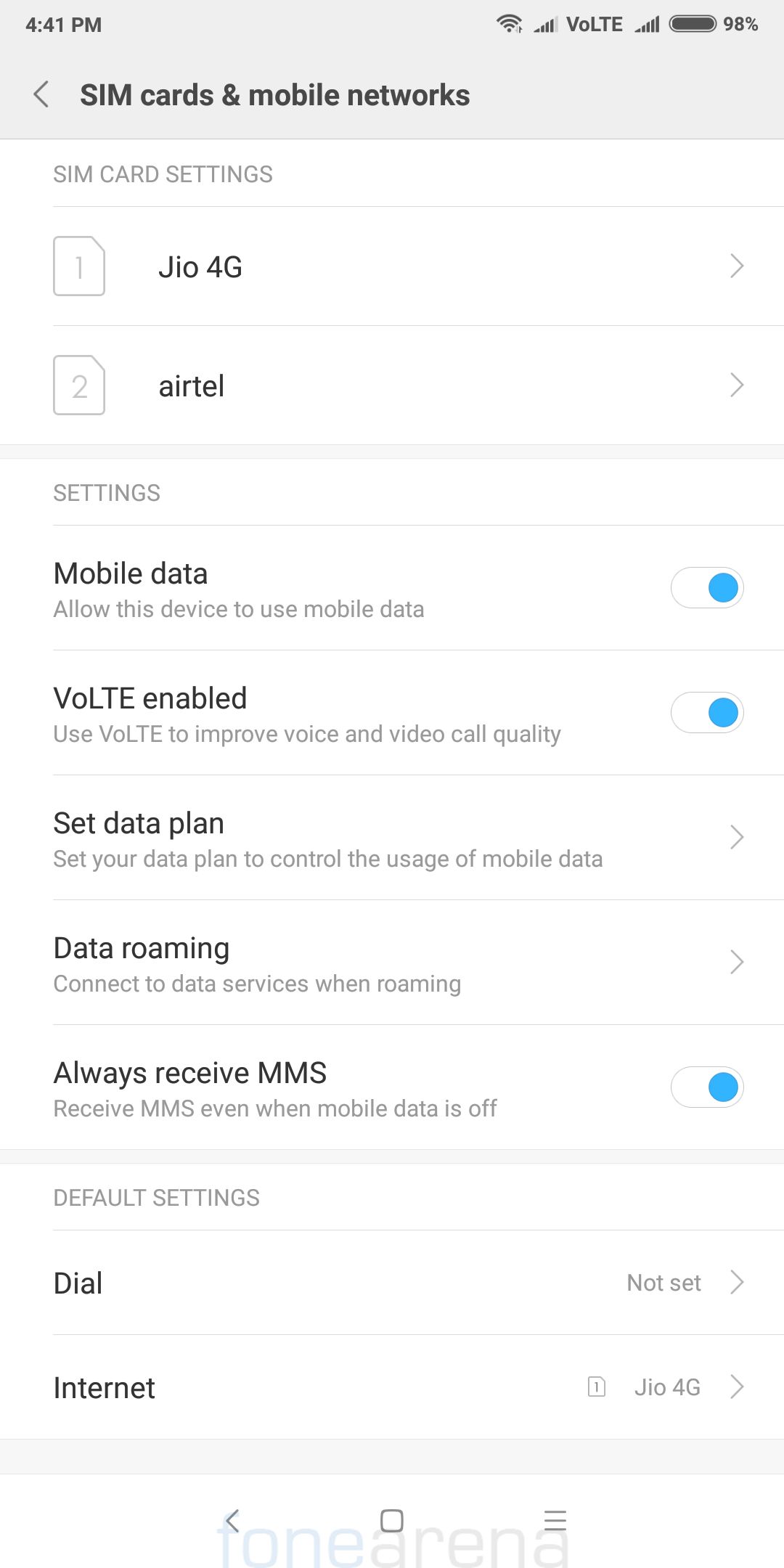A detailed caption for the described image could be:

---
This is a screenshot of the SIM card and mobile network settings from a mobile phone. The screenshot, watermarked with "phonearena" at the bottom in two distinct colors—F-O-N-E in blue and A-R-E-N-A in gray, provides a comprehensive view of the network configuration options available on the device. 

At the top of the screen, a gray border displays the current time, 4:41 p.m., alongside various indicators including data connectivity, Wi-Fi, and V-O-L-T-E, which stands for Voice over LTE. A nearly full battery icon shows a 98% charge level.

Below the gray border, a left-pointing back arrow is labeled "SIM cards & mobile networks," leading into the detailed settings. The displayed options begin with "SIM card settings," listing two SIM cards: "1. GOJIO 4G" and "2. Airtel," both activated for 4G networks.

Further into the settings, the "Mobile data" section is toggled on, allowing the device to use mobile data. The "V-O-L-T-E enabled" option is also active, purportedly to enhance voice and video call quality. Additionally, users can "Set data plan" to manage data usage, toggle "Data roaming" to connect to networks while traveling, and ensure they "Always receive MMS," even when mobile data is off. Lastly, the "Default settings" indicate that dialing is not set, but the internet is configured to "G-O-4-G."
---